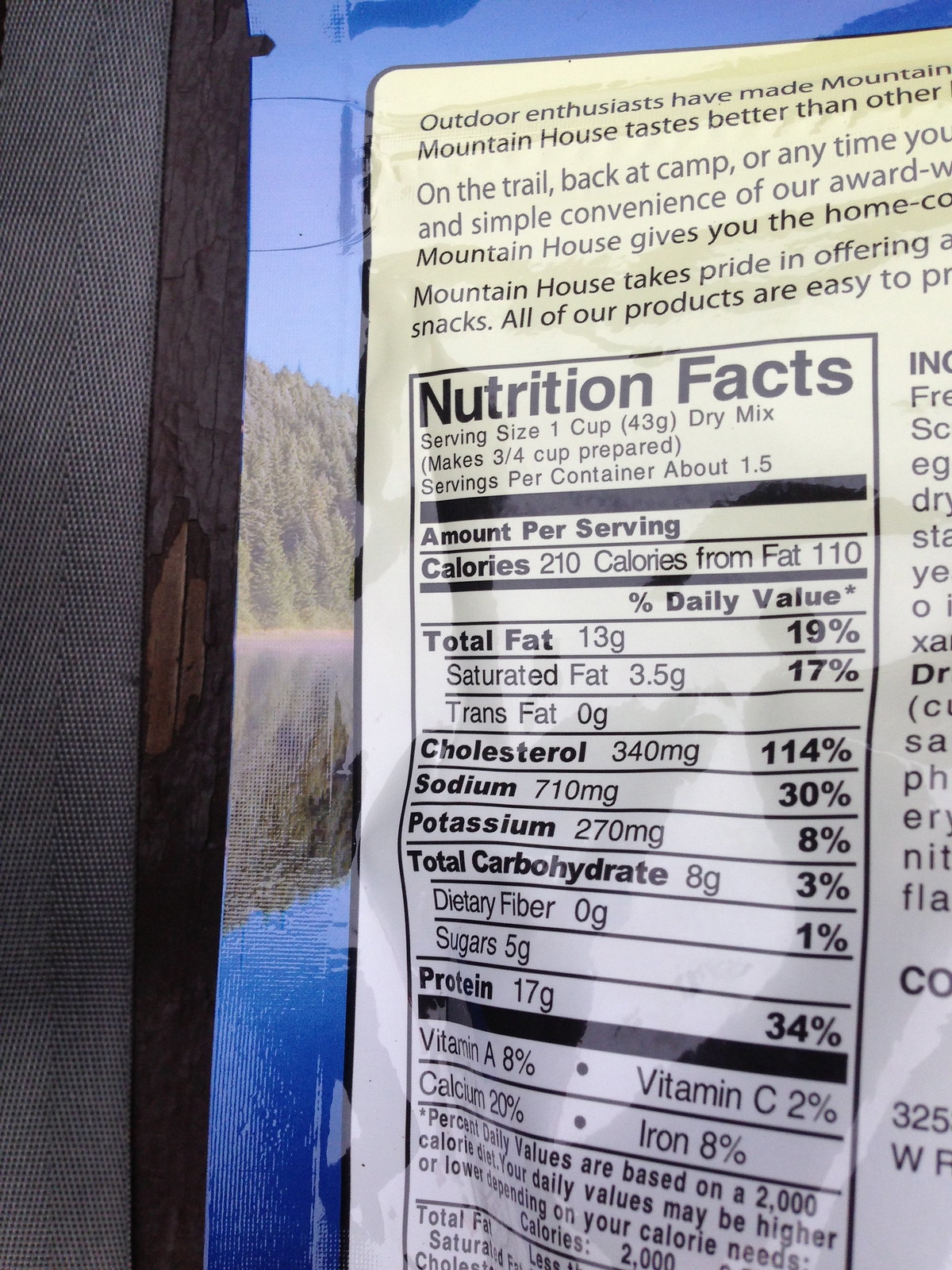This is a detailed close-up photograph of a food packaging for Mountain House products. The packaging features a blue border with a central image showcasing a serene body of water reflecting a tree line, which extends into the background with a clear sky. The bottom part of the package includes a white rectangular section with nutritional facts. The visible portion indicates a serving size of one cup (43 grams dry mix), yielding about three-quarters of a cup when prepared, with approximately one and a half servings per container. Each serving contains 210 calories (110 from fat), 13 grams of fat, 3.5 grams of saturated fat, 8 grams of carbohydrates, 270 milligrams of potassium, and 710 milligrams of sodium, along with 6% of the daily value of Vitamin A and 20% of Calcium.

Surrounding the nutritional facts is a descriptive text emphasizing Mountain House's commitment to convenience and taste, appealing to outdoor enthusiasts whether on the trail, back at camp, or at any other time. The packaging also includes a mission statement in black lettering, affirming the brand's pride in its offering of snacks and meals. The image captures parts of the surrounding environment, showing a light brown fabric and a chipped wooden surface to the left. The scene suggests the product's rugged, outdoor-oriented branding while highlighting the practical information needed by consumers.